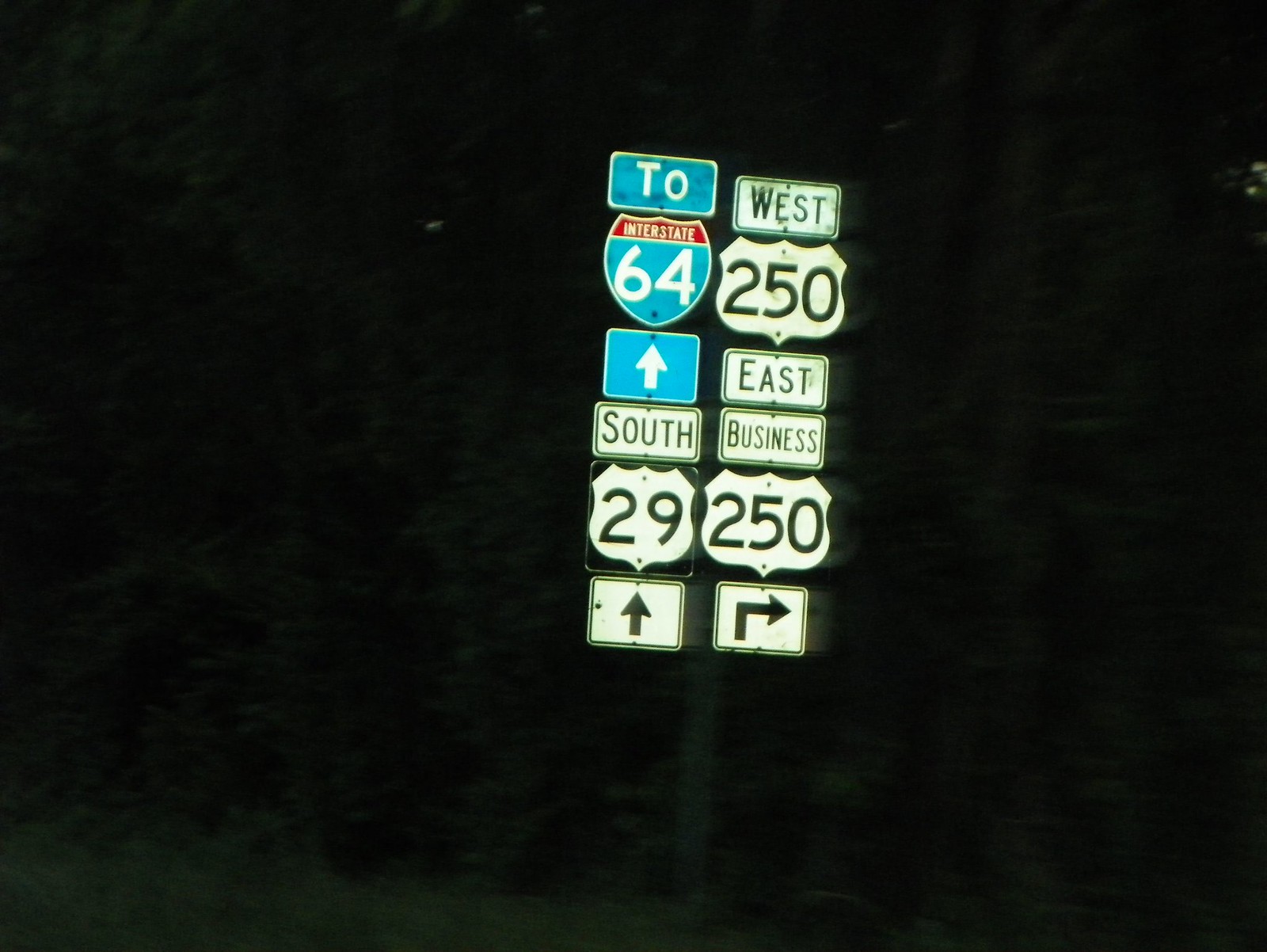This nighttime photograph captures a cluster of illuminated street signs mounted on a single gray pole, positioned along the side of a road, with dark trees forming the backdrop. At the top left of the pole, there is a turquoise sign with white lettering, accented by a red banner. The sign reads "To Interstate 64" with an upward-pointing arrow, indicating a straight-ahead direction. Adjacent to this, on the right, is a black and white sign featuring "West 250 East Business" to denote highways 250, with an arrow pointing to the right for East Business 250. Below the Interstate 64 sign, there is another sign that says "South 29" in black text on a white background, also directing straight ahead with an upward-pointing arrow. This intricate assembly of signs provides guidance for several highways, including an interstate and business routes, amidst the obscurity of the nighttime setting.